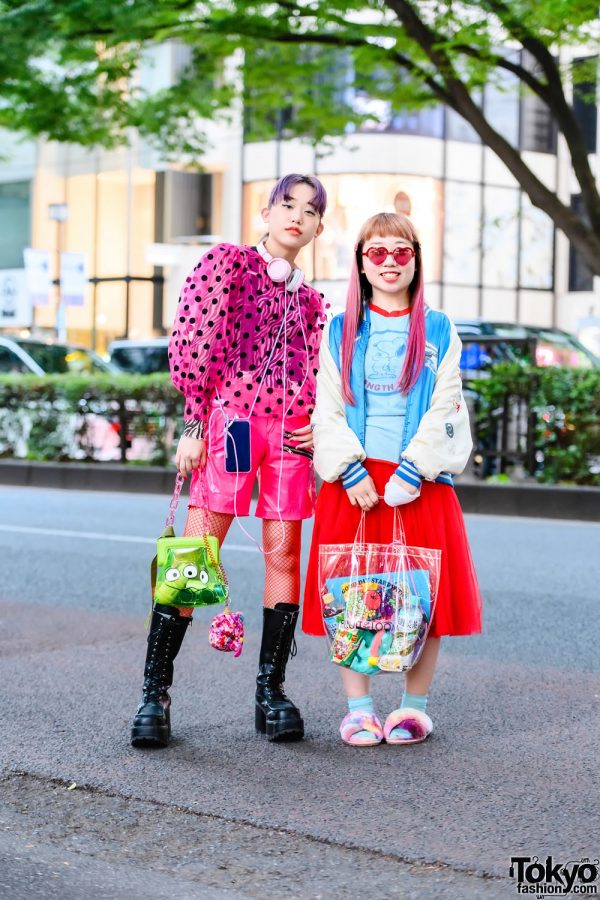Two stylish individuals are posing on a sidewalk, with a clear logo "tokyofashion.com" at the bottom of the image. The person on the left is dressed in a striking outfit featuring a pink shirt with black dots, pink pants, very high black boots, and thick leather shoes with laces. They accessorize with a lime green bag adorned with monster eyes, a phone tied to their pants, headphones, and sport short purple hair. On the right stands another person wearing a blue shirt, a white jacket, a red skirt, furry sandals, and heart-shaped pink sunglasses. They have pink highlights in their hair and hold a clear bag. The background showcases a lively city scene with blurred buildings, a tree filled with green leaves and branches, and some visible automobiles. The lower section of the image displays grey bits with red markings, and green bushes are noticeable behind the duo.